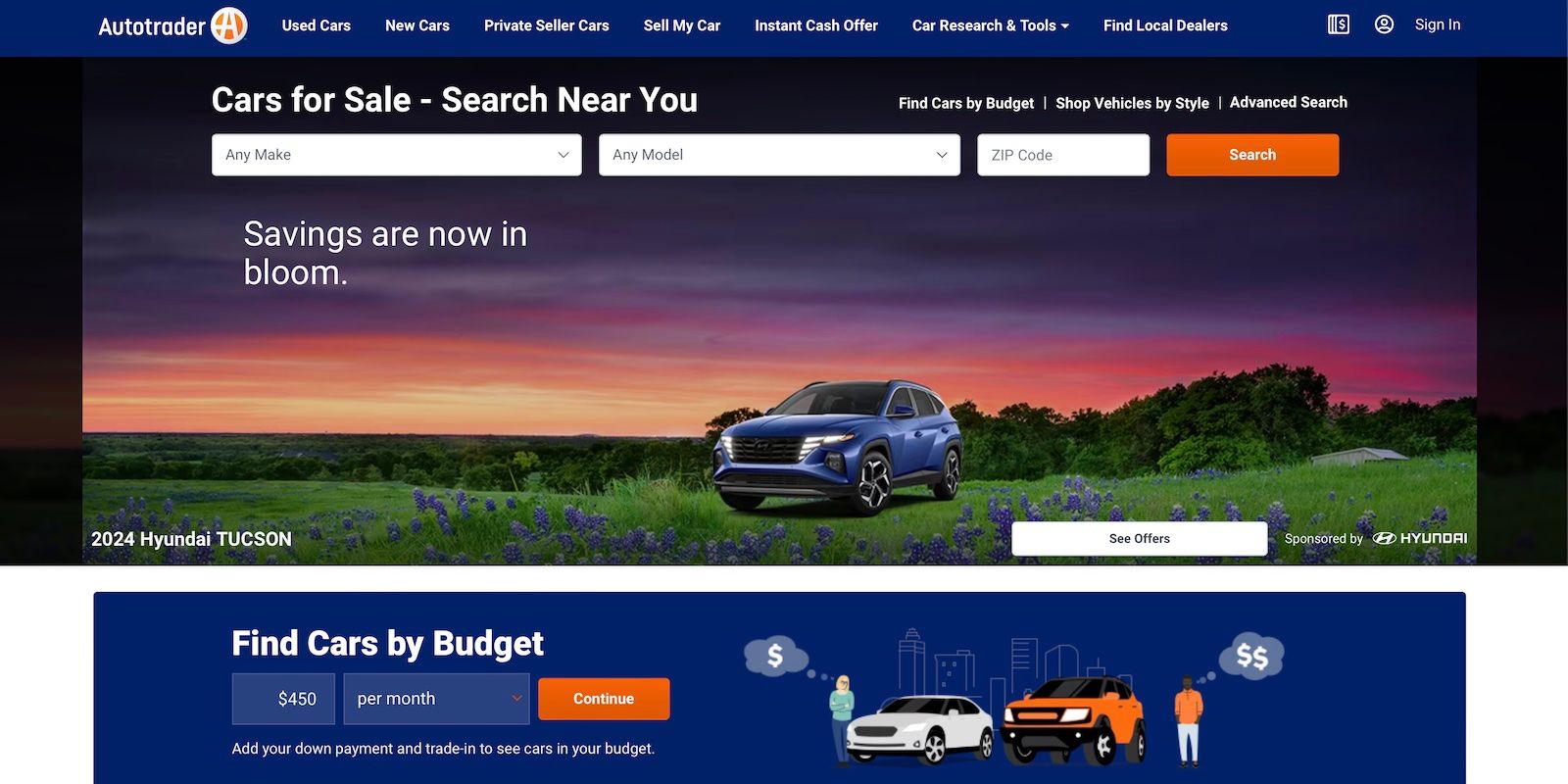The webpage header features the AutoTrader logo, with a distinctive white and orange "A" and "AutoTrader" written in white on a blue background. The header includes several white tabs labeled: "Used Cars," "New Cars," "Private Sale," "Seller Cars," "Sell My Car," "Instant Cash Offer," "Car Research and Tools," and "Find Local Dealers." There is also a cash sign, a "Sign In" button, and a profile icon.

In the central section of the page, on the left, the text reads "Cars for Sale, Search Near You." On the right, the offerings include "Find Cars by Budget," "Shop Vehicles by Styles," and "Advanced Search." Below this, a search module is divided into three sections: "Any Make," "Any Model," and "Zip Code," with an orange "Search" button to the right.

Beneath the "Any Make" section, there’s an advertisement banner stating "Savings Are Now in Bloom," featuring an image of a 2024 blue Hyundai Tucson. The car is parked on green grass surrounded by purple lavender flowers, with green trees and a sunset sky that includes yellow, purple, and dark hues. On the bottom right of the image, a white "See Offers" button appears, accompanied by "Sponsored by Hyundai."

Further down the page, there's a section titled "Find Cars by Budget," promoting vehicles available for $150 per month. An orange "Continue" button is located below, with a prompt underneath advising users to add their down payment and trade-in values to view cars within their budget.